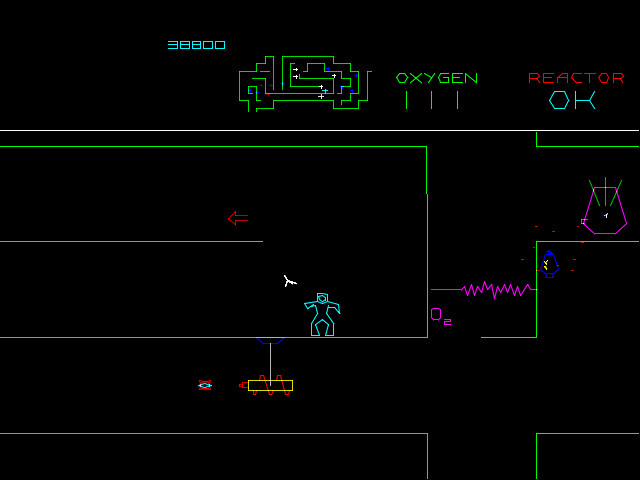This image is a snapshot from a retro-style video game, characterized by its predominantly black background and minimalist digital graphics. At the top of the screen, the score is displayed in blue text, indicating 38,800 points. Next to it, green text reads "oxygen," along with three green bars denoting a full supply. Adjacent to this, "reactor" is written in red text, with a blue icon below it—a blue hexagon and a few blue lines resembling a stick figure lying on its right side, where the hexagon forms the head and the lines form the body.

A zoomed-out, full-size map of the game level is also visible at the top, providing an overview of the maze-like environment. The maze itself is composed of thin, bright green lines that outline various obstacles and platforms. Within the maze, the primary character—a blue, humanoid figure—navigates through the intricate pathways. Scattered throughout are additional elements, including purple enemies, red directional arrows guiding the player, and a yellow rectangular gun with a red barrel.